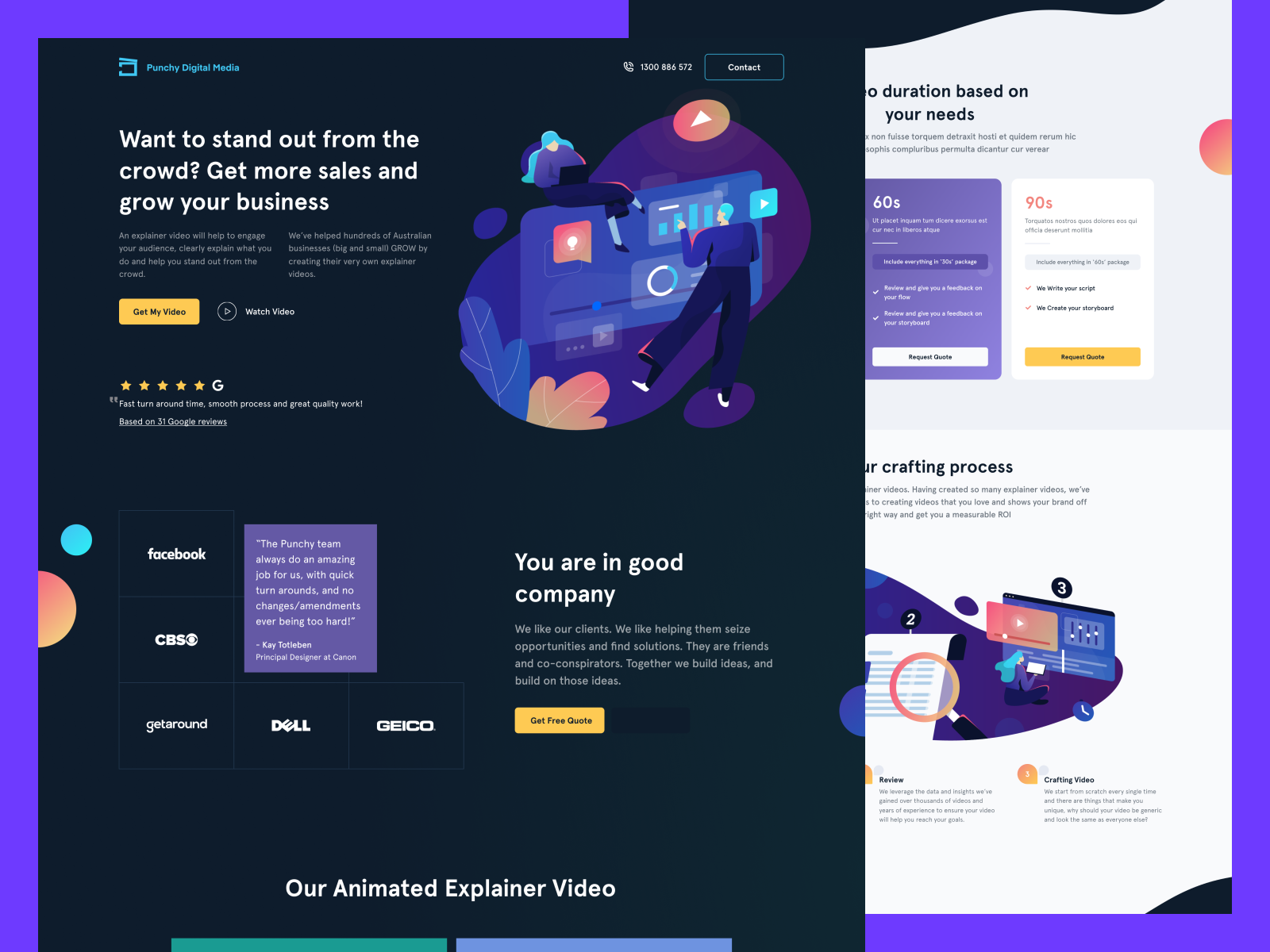This brochure features striking purple edges surrounding a stylish black and white interior. On the black section, bold text announces "Punchy Digital Media" followed by a compelling call to action: "Want to stand out from the crowd, get more sales, and grow your business." Highlighted in an orange box, the phrase "Get the Video" urges engagement, supported by another prompt: "Watch Video."

The brochure proudly showcases five-star accolades, emphasizing a fast turnaround time, smooth process, and high-quality work based on 31 Google reviews. A playful illustration depicts a cartoon man intently working on a large board, while above him, a woman with aqua hair relaxes, either reading a book or using a computer. The background is adorned with artistic elements, including partial gold and blue leaves.

Testimonials add credibility, with notable endorsements: "The Punchy team always do an amazing job for us, with quick turnaround and no changes or amendments ever being too hard," reflecting their work for prestigious clients like Geico, Dell, Getaround, CBS, and Facebook. 

A statement of values follows: "You are in good company. We like our clients. We like helping them seize opportunities and find solutions. They are friends and co-conspirators. Together we build ideas and build on those ideas." The brochure concludes with a call to action, inviting potential clients to "Get a free quote."